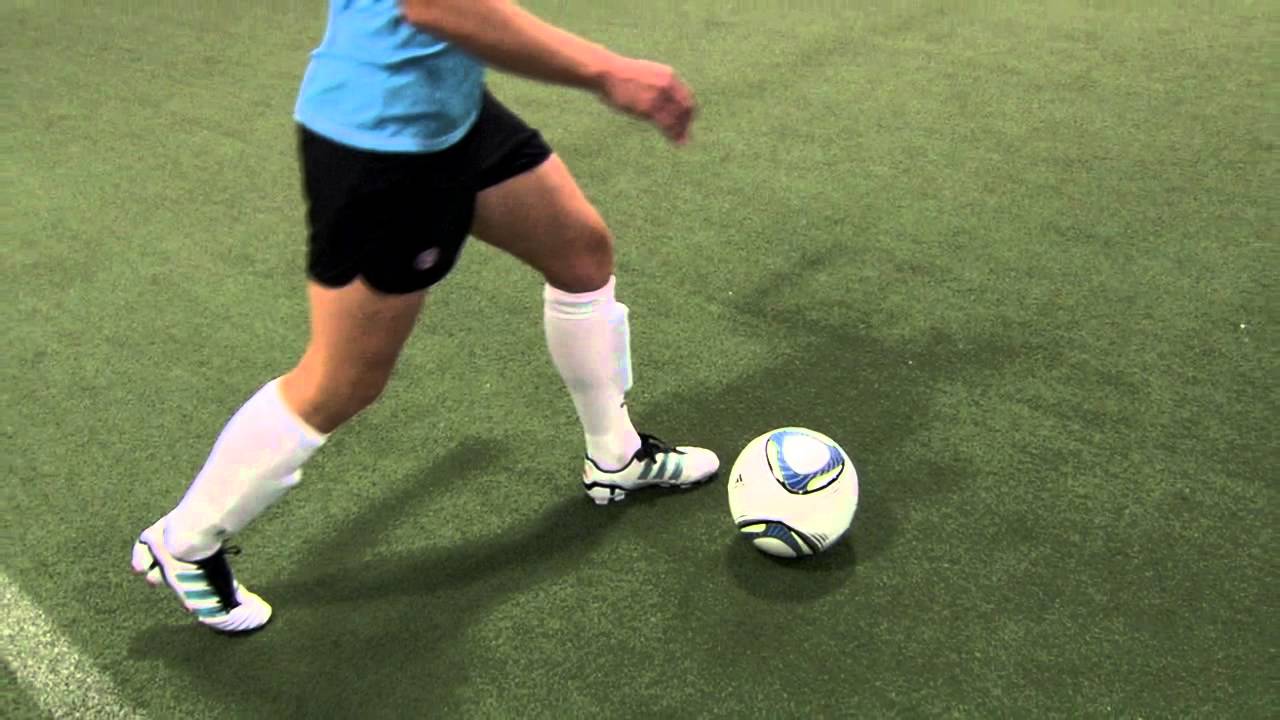The image is a detailed landscape-oriented photograph capturing a dynamic moment in a soccer stadium. The grass surface, which could either be real grass or astroturf, spreads across the bottom of the image. In the lower left corner, a faint white chalk line marks the field. On the lower right, a soccer ball made of white with blue, black, and green circular designs rests on the ground, both the ball and the person casting discrete shadows.

The photograph's main focus is a player, potentially a man, visible from just above the waist to his feet, lunging forward, preparing to kick the soccer ball. The individual appears to be Caucasian and is dressed in a blue top paired with black shorts. The player’s athletic apparel includes white socks that rise just below the knee, encasing shin guards, and white cleats featuring black laces and Adidas’ signature three black stripes.

The player's right arm is poised in front of him, bent at the elbow, lending a sense of movement as he faces and advances towards the right side of the frame, with his left foot forward and his right foot positioned to strike the ball.